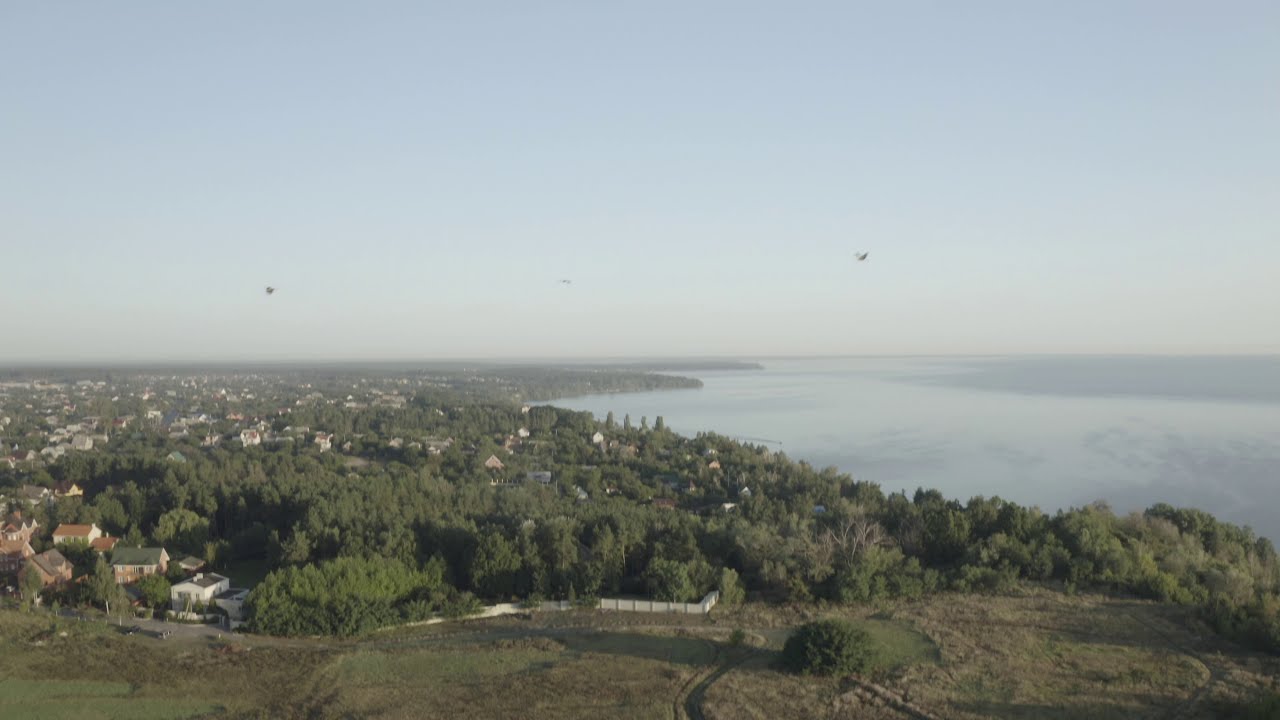The photograph is a horizontally rectangular, slightly faded outdoor image taken during the daytime from an elevated vantage point, possibly from an aircraft. The scene is dominated by a serene blue sky and an expansive blue body of water, likely a large lake or the ocean, which occupies the right side of the frame. At the bottom of the image, a lush green field stretches out, blending into a dense area of vividly green trees. Scattered among the foliage are numerous small homes, particularly congregated toward the left side of the image. The colors in the photograph range from light blue, green, and brown to hints of white, yellow, orange, tan, and black. The entire ensemble appears to be a tranquil aerial view of a small town situated amidst natural surroundings.